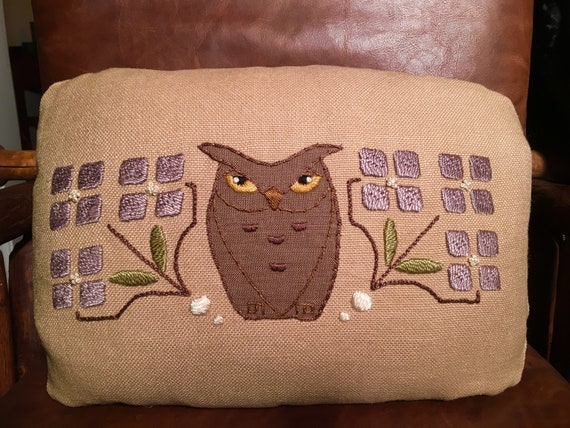This image captures a decorative pillow placed on a leather office chair, which is only partially visible. The chair, made of brown leather with tan wooden handles, provides a warm backdrop for the pillow. The pillow itself is crafted from a tan, burlap-like fabric and features an intricate embroidered design. Central to the pillow's decoration is a brown owl with yellow eyes and a brown beak, encased in a shield-like outline. Surrounding the owl, symmetrical patterns of four brown indentations and twelve small white balls—arranged in a grid of 24 squares, twelve on each side—enhance the design. Additionally, green leaves with stems intricately frame the owl, adding a touch of nature to the overall aesthetic. The portrayal of the owl with slightly angry eyes adds character and depth to the artwork.